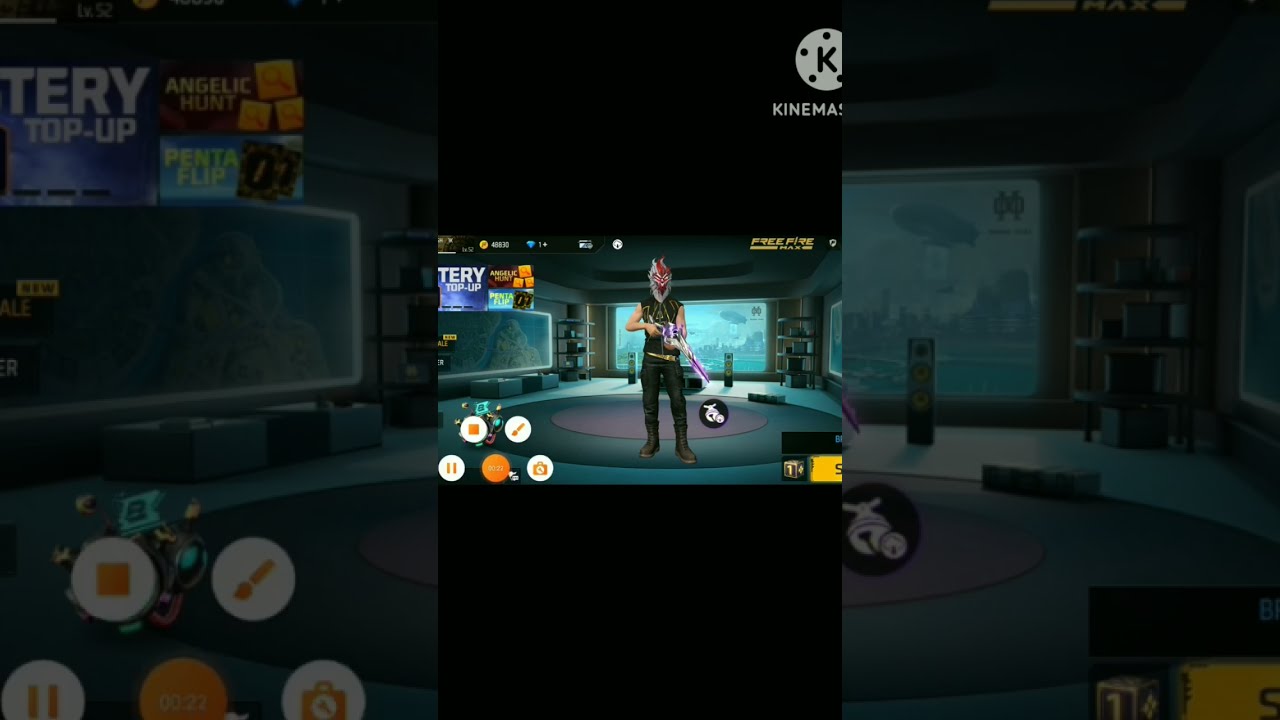The image appears to be a composite screenshot from a video game, meticulously divided into three vertical sections. The central third features the main image, while the left and right thirds display zoomed-in, blurrier portions of the central image. The central part of the picture itself is segmented horizontally into three parts: the top and bottom thirds form plain black borders. 

At the top border, a white circle encases a black 'K' and several black dots, followed by the partially visible text "K-I-N-E-M-A-S," indicating potential branding or title information. Below this, the key image portrays a male video game character standing in a room with large screen displays in the background. The character, likely of Caucasian descent, is outfitted in dark jeans, black boots, and a sleeveless black top, with a peculiar white and red mask resembling a cross between a Muppet and a chicken. His right hand wields a glowing purple and white gun.

The background features recognizable elements such as large window-like screens and a circular rug that resembles a vinyl record. In the bottom left corner of the central image, there are visible on-screen controls, including icons such as a pause button, a camera, and an unclear additional option. The visual details create an impression of a selection or customization screen within the game.